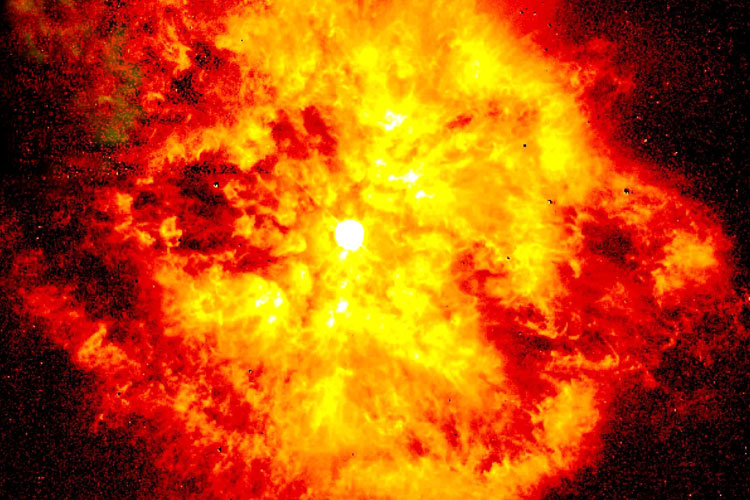This digital image depicts a massive explosion, likely in space, resembling a supernova—a colossal stellar explosion following the collapse of a sun. At the very center lies a small, intense white core, surrounded by a bright yellow nucleus that diffuses into deep oranges and dark reds, all radiating outward in a spectacular burst. The surrounding black background enhances the explosion's vivid colors, contrasting sharply with the fiery display. The explosion extends to the edges of the image, filling the frame with splashes of yellow, orange, and red, accented by thick clouds and smoke, which emphasize its vastness and complexity. Particles dot the scene, adding texture and depth, while areas of concentrated color intermingle with the dark void, creating an otherworldly, almost surreal dynamic.